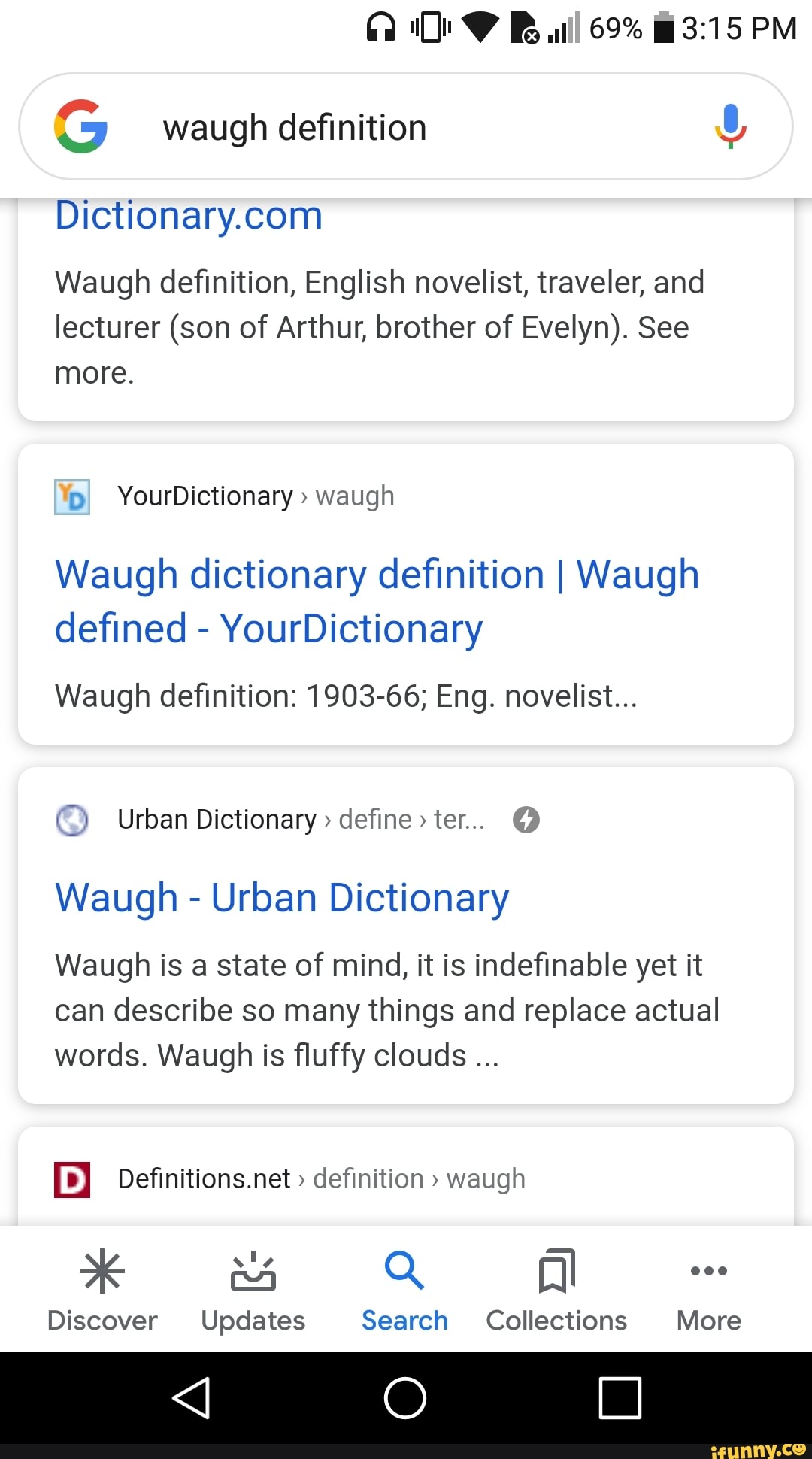This image appears to be a screenshot taken from a person's smartphone, capturing their internet browsing activity. The top right-hand corner of the image displays several phone status indicators: a signal bar indicating network connectivity, battery life percentage, an icon showing that headphones are connected, and a vibration symbol confirming that the phone is on silent mode. 

The main content of the screenshot is a web browser search using Google. The user has typed "WAUGH" into the search bar, looking for its definition. The search results show multiple options for what "WAUGH" could mean, including links from Dictionary.com and U Dictionary. The Dictionary.com entry suggests that WAUGH may refer to an English novelist, traveler, or lecturer, specifically noting relations to the author Evelyn Waugh. Further options from general dictionary databases provide various definitions and contextual uses, though some information is cut off by the constraints of the screen.

At the bottom of the screen, there are several navigation options available within the app, including "Discover," "Updates," "Search," "Collections," and a "More" menu, likely offering additional features and settings.

Overall, this detailed screenshot offers a glimpse into the process of looking up definitions and the interface elements of a mobile web browser.